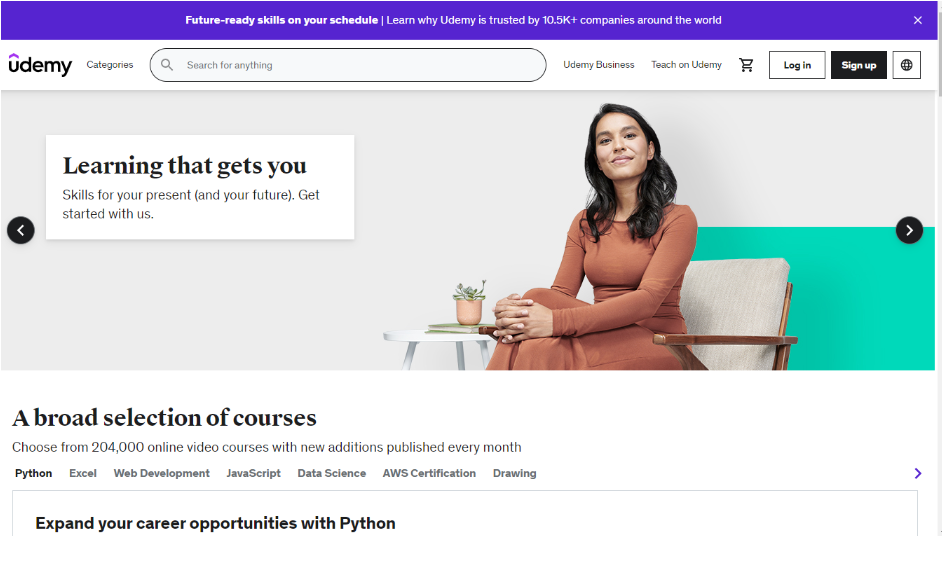In this screenshot of the Udemy login and sign-up page, a purple stripe sits at the very top of the page, proclaiming, "Future-ready skills on your schedule." Below this, there's a banner reading, "Learn why Udemy is trusted by 10.5k+ companies around the world." The navigation bar includes the Udemy logo, categories, a search bar, and options for logging in and signing up.

Prominently featured on the right side of the page is a woman with medium-dark skin, dressed in a tight-knit dress. She has dark hair, a bright smile, and an expression of pride. She is seated on a plain chair with a cushion, her legs crossed and hands folded over her raised knee. Next to her, there is a small table adorned with a modest plant.

The text accompanying the image states, "Learning that gets you. Skills for your present and your future." It encourages visitors to "Get started with us," highlighting "a broad selection of courses" and adding, "Expand your career opportunities with Python."